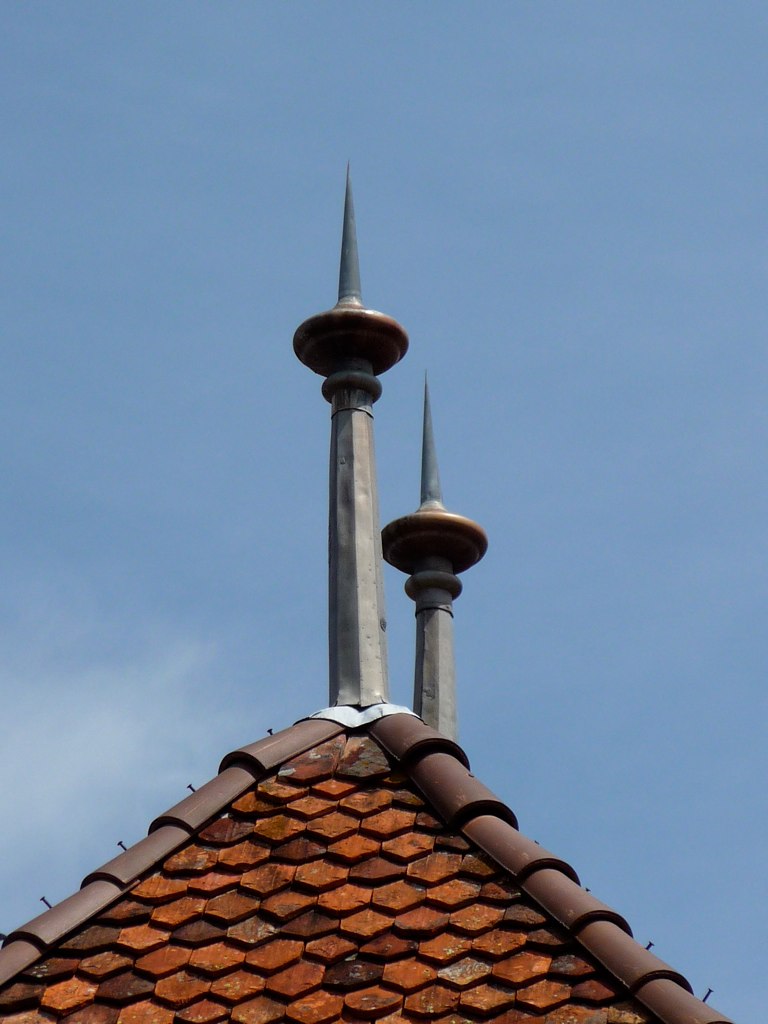The image captures the peak of a roof covered with small, burnt orange and dark brown shingles. Atop the roof, two prominent metal structures rise into sharp, thin points. These structures are layered and characteristic, with a base that tapers up into a spiked end, adorned with circular elements halfway up. The structures create a symmetrical visual, with one positioned directly at the triangular peak of the roof and the other slightly behind it. This detailed roof scene is accentuated by the light blue sky above, with a wisp of a white cloud visible on the left side, adding a serene backdrop to the striking architectural features.